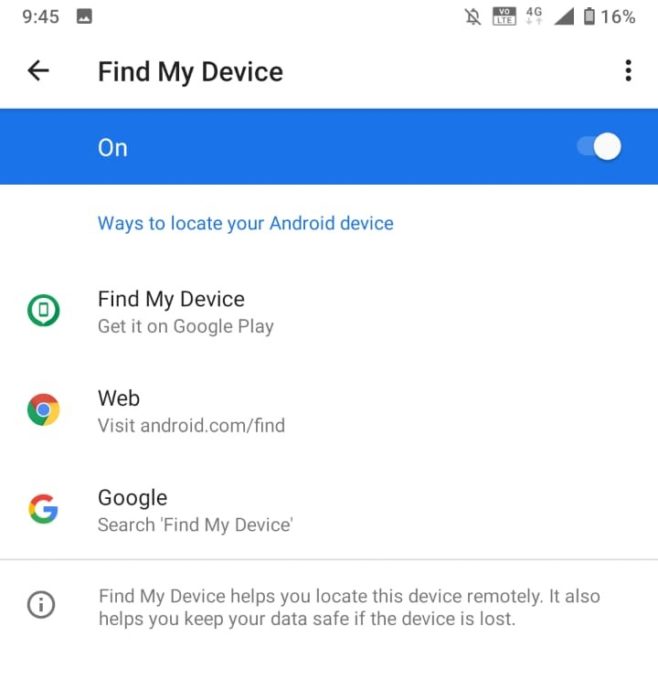This screenshot from a cell phone or tablet shows a detailed interface related to the "Find My Device" feature. In the top-left corner, the time is displayed as 09:45, possibly in military time format since no AM or PM is specified. Next to the time, there is a screenshot icon characterized by a black square with a white mountain range, and a bell icon with a line through it indicating that sound is muted.

Next, a square labeled 'VO' is seen, with a black upper half and a split lower portion showing 'LTE.' Following this, '4G' is shown along with up and down arrows to indicate data speed. On the top right, a full signal strength bar is visible, and next to it is a nearly empty battery icon showing 16% remaining battery life.

Within the same white area and on a new line, there is a dark black left-pointing arrow, followed by bold black text that reads "Find My Device." To the right, three ellipses indicate more options. Below this, a dark blue rectangle contains the word 'ON' in white, accompanied by a mid-blue slider with a white circle on the right side.

Underneath in another white area, it shows "Ways to locate your Android device" in blue. Below this, a green circle with a green phone icon is shown inside a white area, labeled "Find My Device" in bold black text. Under this, gray text reads "Get it on Google Play," accompanied by the Google Chrome symbol, which consists of sections in red, green, and yellowish-orange creating a circular shape around a blue center with a thin white ring.

Below this is the URL "visit android.com/find," in bold black text. Further down, the Google logo is displayed with a multicolored 'G' transitioning from red, to yellow-orange, to green, and then blue. This is followed by 'Google' in bold and 'Search "Find My Device"' in gray.

Continuing, an information icon—depicted as a black 'i' inside a circle—is followed by gray text that explains, "Find My Device helps you locate this device remotely. It also helps you keep your data safe if the device is lost."